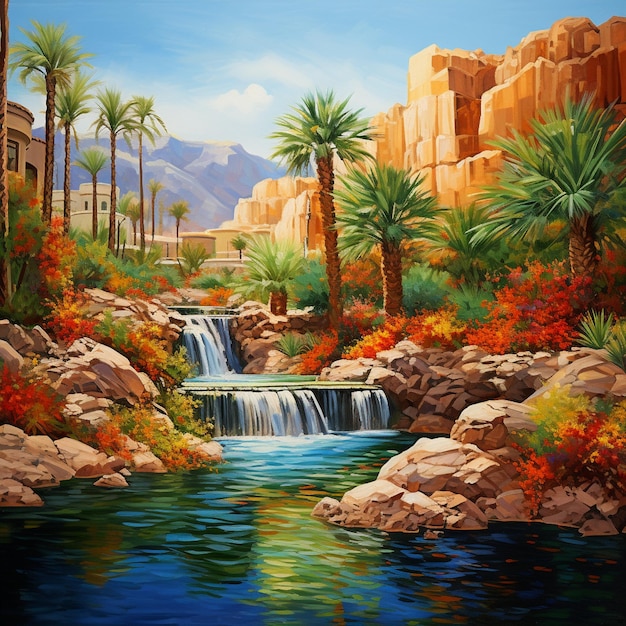The image showcases what appears to be a digitally created artwork that captures a vibrant and serene natural scene. At the bottom, there is a small lake reflecting lush colors from the scenery above, particularly greens and reds. This lake leads to a cascading waterfall at the center, which flows into another waterfall further behind.

On both the left and right sides of the lake, rocky outcrops adorned with red and green plants are visible, as well as palm trees growing along these rugged terrain features. A series of buildings is partially obscured by the palm trees on the left, adding a touch of human presence to the setting. Further back, the scenery transitions into modestly tall, stone cliff sides on the right and a blue-tinted mountainside beneath the clear sky on the left.

The top of the image showcases a bright blue sky dotted with white clouds, complementing the scene with ample natural lighting. This detailed representation combines natural elements like cliffs, rocky outcrops, trees, and waterfalls, unifying them in a harmonious and colorful landscape.